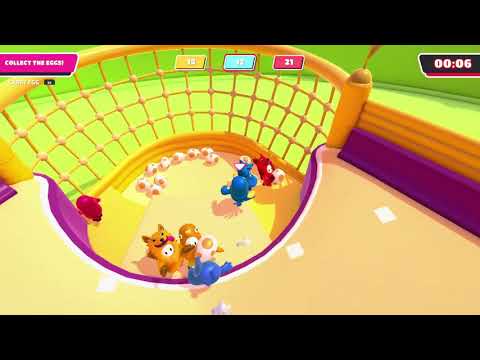The image is a detailed scene from a colorful video game. Central to the image is a convex arena, resembling a pocket of a pool table, framed by a light orange net with webbed circles and bordered by purple edges. The arena floor is a light cream or beige color, dipping downward into the netted area. Inside the arena pit are several cartoonish 3D animal characters, which are brightly colored and bubbly in shape, including figures like a dog and an orange cat with its tongue sticking out, as well as characters in blue, red, and orange. Scattered around on the ground are white balls or eggs with light tan spots. The background of the image has a lime green tone, adding to the game's playful aesthetic. At the top center of the screen, there are numbers indicating scores, and at the top right, a black rectangular timer shows "00:06". To the left, a pink highlighted bar reads "collect the eggs," emphasizing the game's objective. The overall color scheme is pastel and childlike, with an emphasis on bright, soft tones.